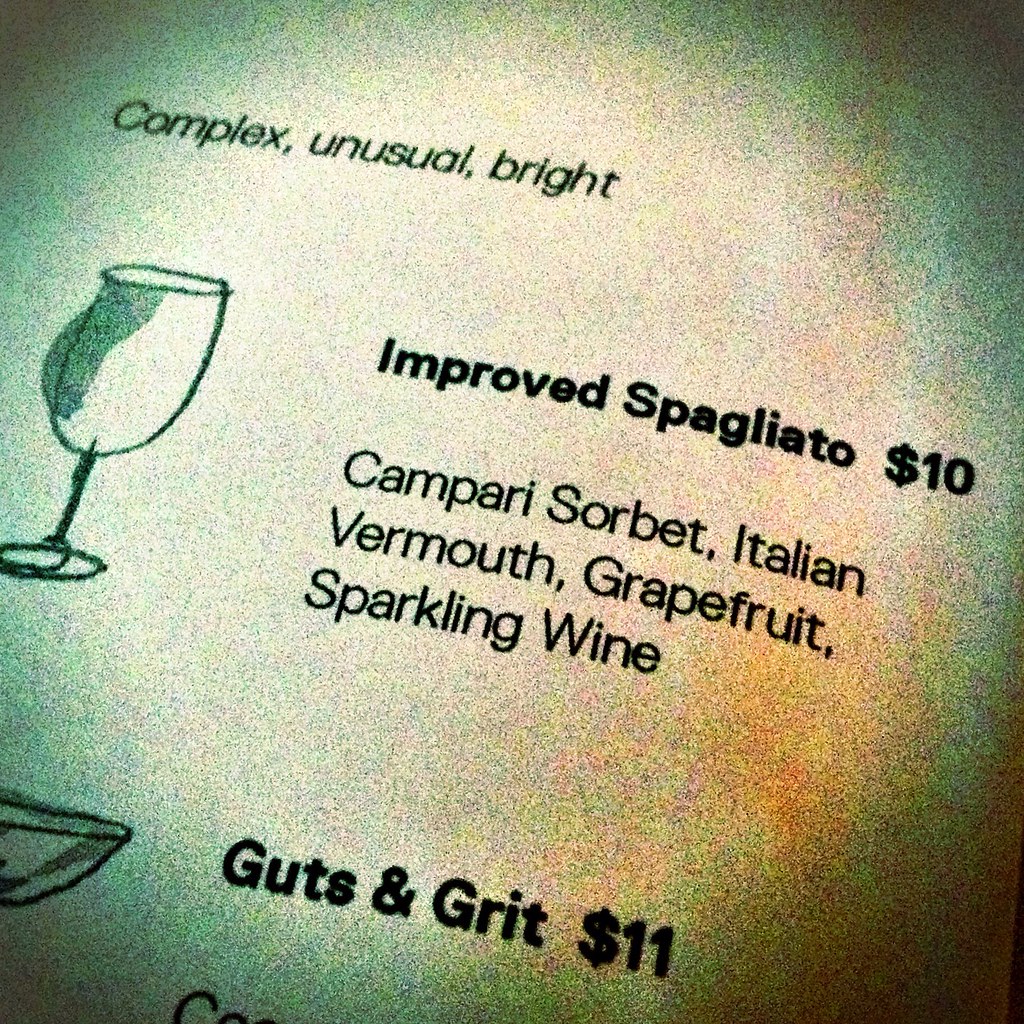The image is a square, close-up photograph of a menu with a vibrant, modern aesthetic. The background is a gradient that transitions from dark green at the edges to bright yellow and orange in the center, creating a marbled effect.

On the upper left side of the image, there are two illustrative drawings. The top drawing depicts a wine glass with shading on its left side, and beneath it is a sketch of a very thin bowl, also with some shading.

In the top left corner, text reads "Complex Unusual Bright." To the right of the wine glass drawing, the menu item "Improved Spagliato" is listed, priced at $10. The description underneath includes the ingredients: "Campari Sorbet, Italian Vermouth, Grapefruit, Sparkling Wine."

Below this, near the drawing of the thin bowl, there's another menu item titled "Guts & Grit," priced at $11.

The image is arranged in two distinct columns: the left column features the illustrations, while the right column contains the descriptions and prices of the drinks. The overall composition is striking due to the marbled background, which enhances the modern and visually appealing design of the menu.